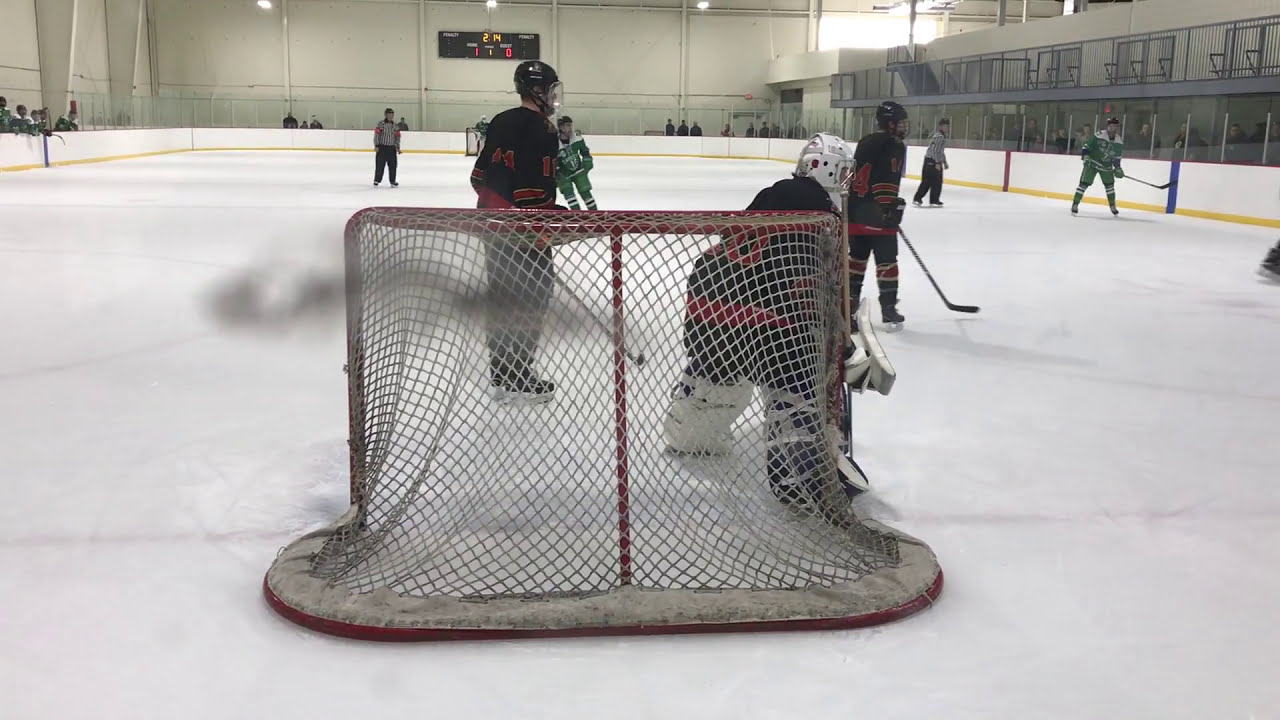This photograph captures an ice hockey game in progress at a modest-sized rink, perhaps belonging to a high school or college. The image is taken from behind one goalpost, providing a clear view of the action. 

In the frame, the goalie, poised and ready to block a shot, stands at the goal, which features a metallic frame and a white net. The two competing teams are distinct in their uniforms: one team in black with red stripes and the other in green with white stripes. The players, equipped with ice hockey sticks and skating on the ice, are intensely focused on the puck.

On the rink, there are referees overseeing the game, adding to the competitive atmosphere. Surrounding the ice are white walls adorned with red, blue, and yellow details. At one end of the rink, a scoreboard displays the time, 2:14, and the score, 1-0, contributing to the game's tension.

Beyond the rink's boundaries, spectators are gathered, closely following the match. Although the arena lacks extensive stands, it accommodates several viewers who are not part of the teams' coaching staff or players. The scene suggests an intense, competitive game in a community-focused setting.